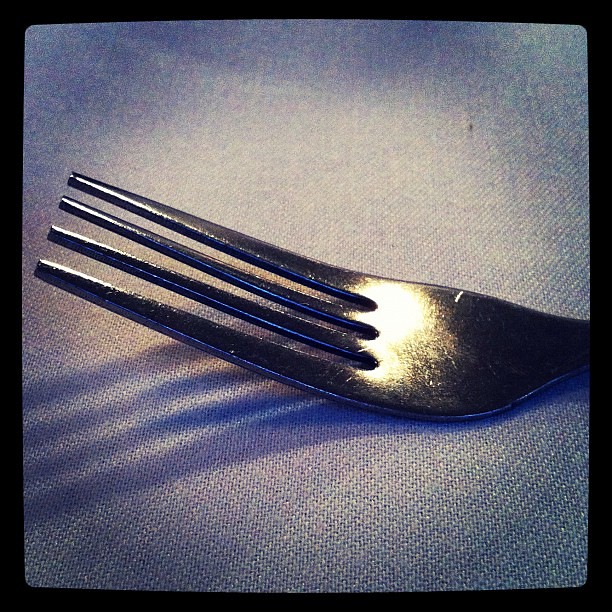This photograph is a highly detailed close-up of a dinner fork, emphasizing its prongs and the intricate weave of the fabric it rests upon. The fork, which is a clean and unused silver, is positioned with its curved side down and its prongs pointing to the left. The image captures the prongs in such detail that even the reflection of the light at their base is visible. The fabric beneath the fork resembles gray denim or a woven tablecloth, which is so finely detailed that the weave pattern is distinctly visible. A light source from above casts a shadow of the prongs on the fabric and creates a lighter spot amidst the darker gray background. The entire scene is framed in black, giving it an artistic, display-worthy appearance.